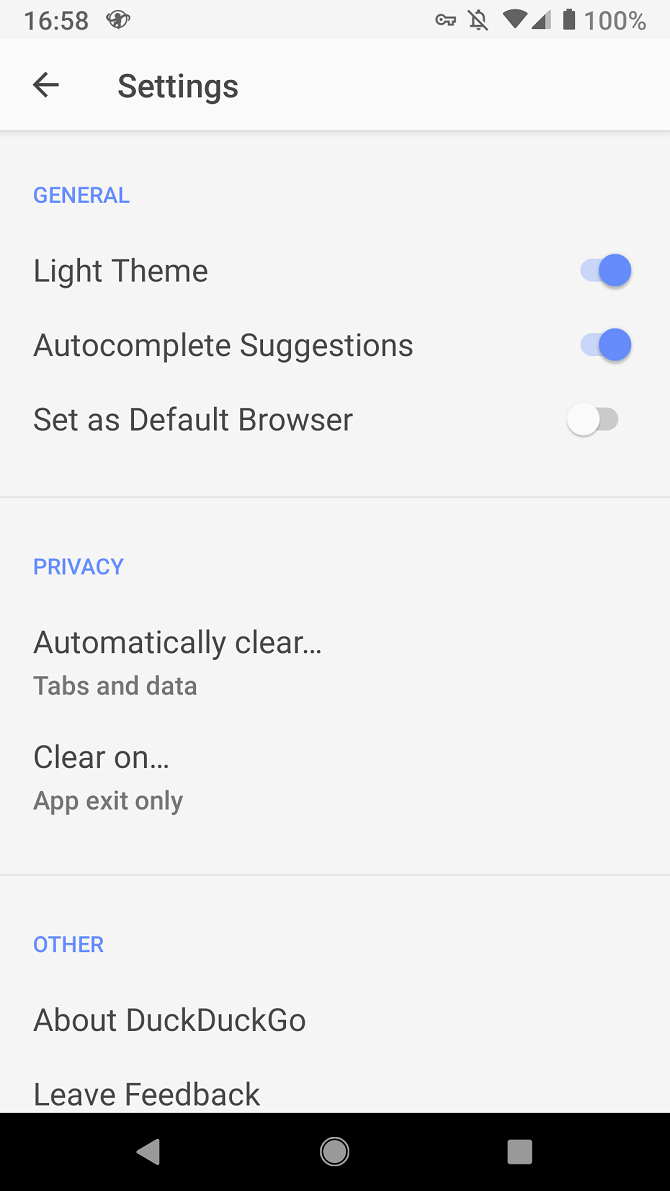The image captures a settings page from a smartphone application. At the top, the banner displays the time "16:58" on the left, followed by an unclear icon. On the right side of the banner, several icons are visible: a key, a bell with a line through it indicating notifications are muted, two triangle shapes, and a battery icon showing 100% charge.

Below the banner, a navigation header features a "Settings" label with a left-facing arrow beside it. The first highlighted section is titled "General" in blue. Under this section, there is an option for "Light Theme" with a slider bar that is engaged and colored blue, indicating it is activated. Next, the "Auto-complete suggestions" option is also turned on, evidenced by its blue slider. The third option, "Set as default browser," has the slider positioned to the left and colored white, meaning it is not activated.

The next main section, labeled "Privacy" in blue, contains settings for "Automatically clear tabs and data" with the condition "Clear on app exit only" specified below it. At the bottom of the settings page, under a section called "Other" in blue, are options labeled "About DuckDuckGo" and "Leave feedback."

The bottom of the image features a black navigation bar with three symbols: a left-facing arrow on the left, a circle in the center, and a square on the right.